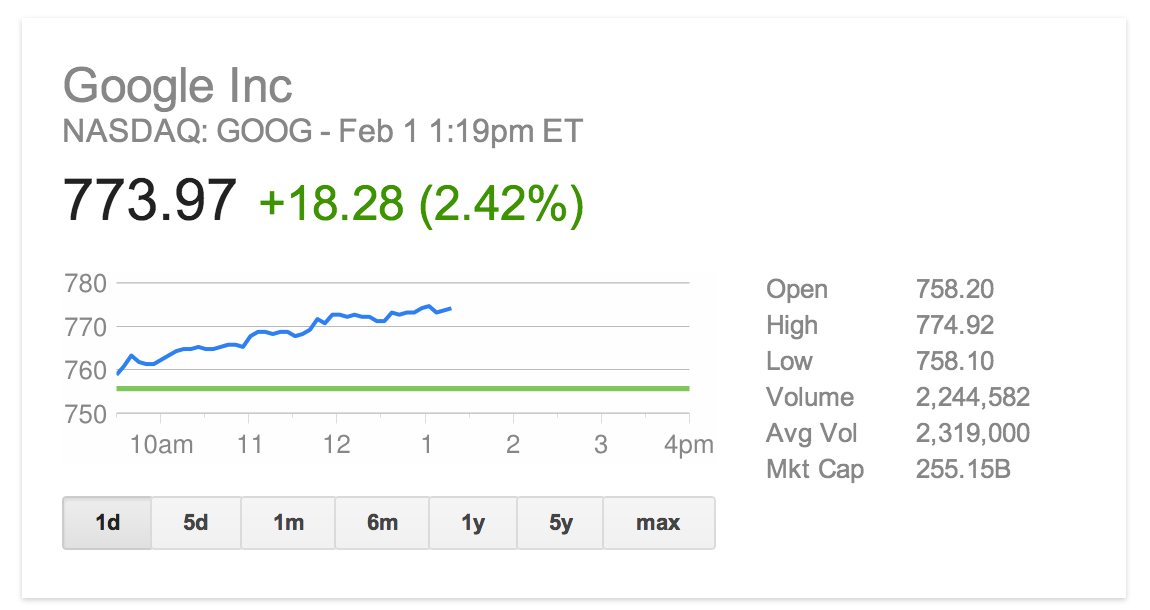The image features a financial chart on a white background with a faint gray border surrounding a large rectangle. At the top, it displays "Google Inc." in gray text, followed by "NASDAQ: GOOG" and the timestamp "February 1, 1:19 PM ET" also in gray. Beneath this, in bold black text, is the current stock price "773.97." To the right of this price is a green plus sign indicating an increase of "18.28" points, or "2.42%" in parentheses.

The chart itself includes price markers at 780, 770, 760, and 750, each indicated by fine gray lines. There's a prominent green line between the 750 and 760 marks, with a blue squiggly line starting at 760 and curving upward, tracking the stock's movement. The bottom of the chart shows a time axis labeled from 10 AM to 4 PM.

A gray banner at the lower part of the image offers different time frame options for the chart display: "1D," "5D," "1M," "6M," "1Y," "5Y," and "Max." 

On the right side, detailed metrics are provided: 
- Open: 758.20
- High: 774.92
- Low: 758.10
- Volume: 2,244,582
- Average Volume: 2,319,000
- Market Cap (MKT CAP): 255.15B